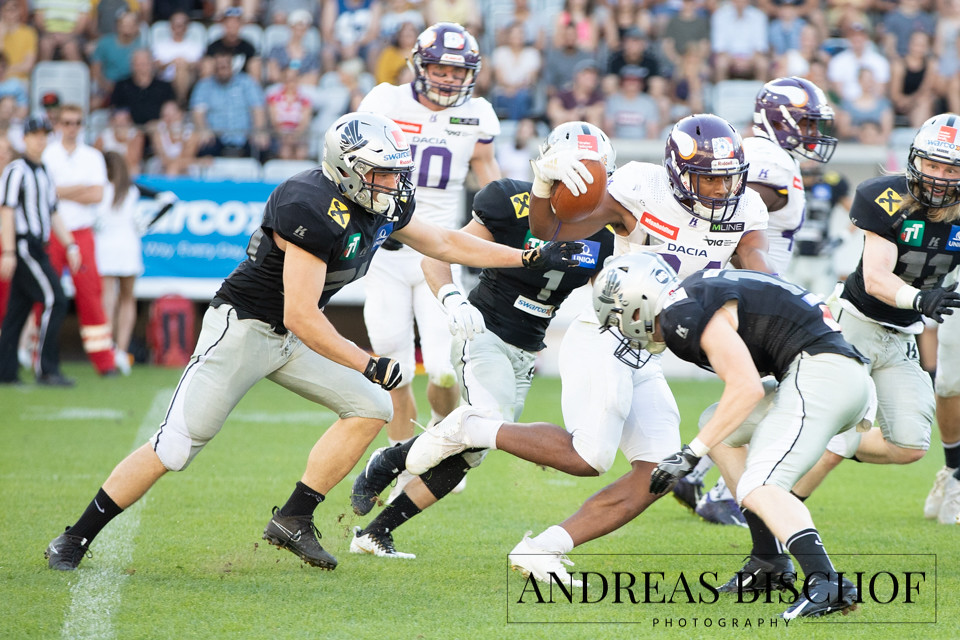This dynamic action shot, captured by Andreas Bischoff Photography, portrays an intense moment in what appears to be a high school American football game. On a lush green field, the game features teams clad in strikingly different uniforms. The team in white jerseys, also identified by the name "Dacia" on their uniforms, sports blue helmets adorned with white wing-like designs. Their opponents, in black and yellow, wear gray helmets with intricate feather patterns.

In the frame, a player from the white team grips the football in his right hand, attempting to push forward. He is braced for impact, as a blue-clad player drives his shoulder into the ball carrier's stomach, while another blue uniformed player closes in from behind, ready to make a tackle. Additional players from the blue team, positioned strategically behind and to the side, prepare to secure the ball in case of a fumble.

The background is a blur of spectators in packed bleachers, adding a vibrant energy to the scene. The referee is also visible, ensuring fair play, amidst the action on the field. Overall, the image encapsulates the energy, strategy, and split-second decisions that define American football.